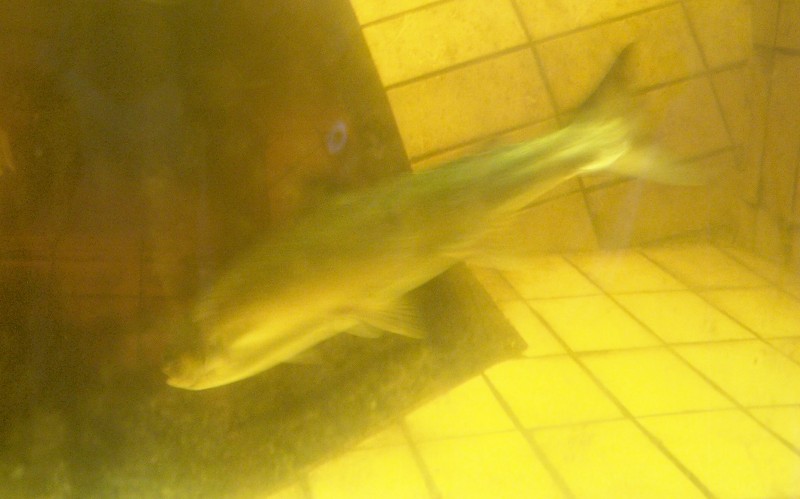This horizontally-aligned, rectangular photograph depicts a single, elongated, and somewhat skinny fish swimming in a murky, yellowish-tinted tank. The fish, resembling a trout, has a silvery appearance with a hint of reddish and greenish hues. The tank is constructed with small, square tiles featuring darker grout, contributing to the overall yellowish tint. The tile arrangement is peculiar, particularly where they meet at off angles in the corners, giving it a non-uniform appearance. In the left portion of the image, occupying roughly a third of the space, an object that resembles a rug or tarp with circular cut-outs hangs into the water, adding to the scene's disarray. Light filters into the water from the right, casting shadows on the left side, particularly where the fish's head is directed, creating a varied illumination across the scene.